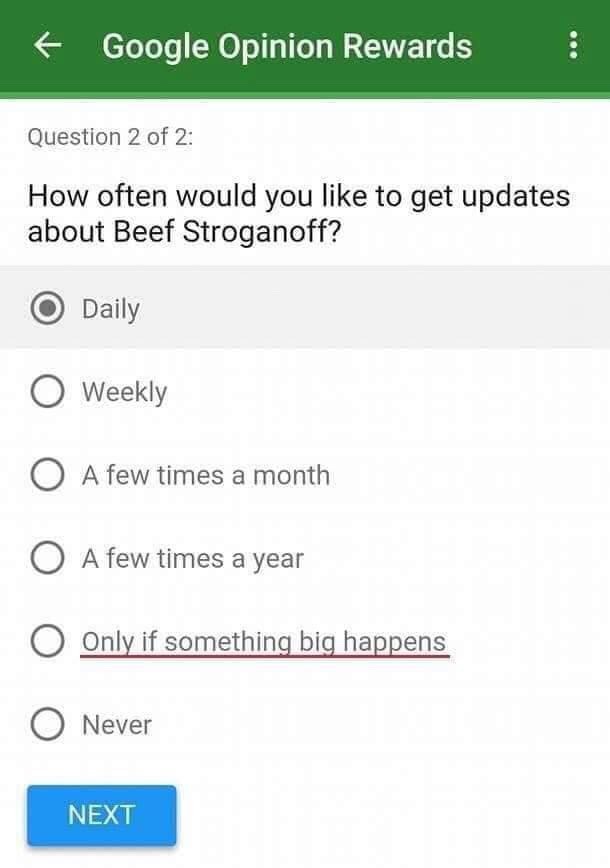This screenshot, resembling a phone or tablet display, prominently features a user interface from the "Google Opinion Rewards" app. At the top, a green header spans across the screen. On the left, an arrow icon points leftwards, next to the "Google Opinion Rewards" text in white. On the right side of the header, there are three vertically-aligned dots symbolizing additional options.

Below the header is the text "Question 2 of 2" in a light font. Beneath this, in bold and slightly larger text, is the question: "How often would you like to get updates about beef stroganoff?" 

A list of six selectable options is presented, each accompanied by a circle. The options are: Daily, Weekly, A few times a month, A few times a year, Only if something big happens, and Never. The option "Daily" is highlighted with a darker gray circle inside a lighter gray rectangle, indicating it has been selected. Below the "Only if something big happens" option, a maroon underline emphasizes this selection.

At the bottom of the screen, a small blue rectangle button displays the word "Next" in yellow letters. The background of the overall interface is white, and the text is in a standard font, with specified parts having contrasting types for emphasis.